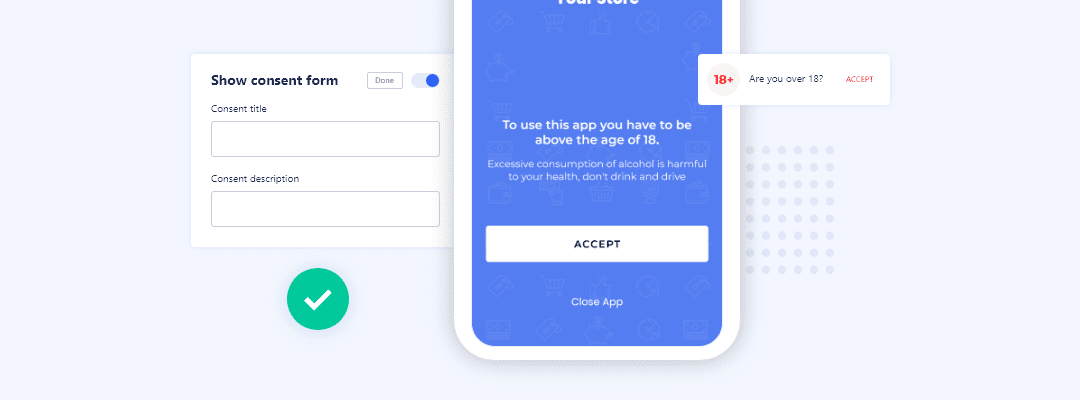The image features a very light blue background. On the left side, there's a compact white drop-down menu labeled "Show Consent Form," accompanied by a small white button that reads "Done." Just below this, there's a small blue circle titled "Consent Title," followed by a text box for the consent description. A green circle with a check mark is also present in this section.

Dominating the center of the image is a larger blue background area. Near the top, only the bottom parts of some white text are visible. The main text within the center states: "To use this app, you have to be above the age of 18. Excessive consumption of alcohol is harmful to your health. Don't drink and drive." Below this message, there is a white button labeled "Accept," alongside another button labeled "Close app." 

Towards the lower part of the image, a small white box contains red text "18+" and a blue question, "Are you over 18?" followed by a red "Accept" button. Faint, indistinct shapes and figures can be seen in the background, adding an element of subtle detail to the scene.